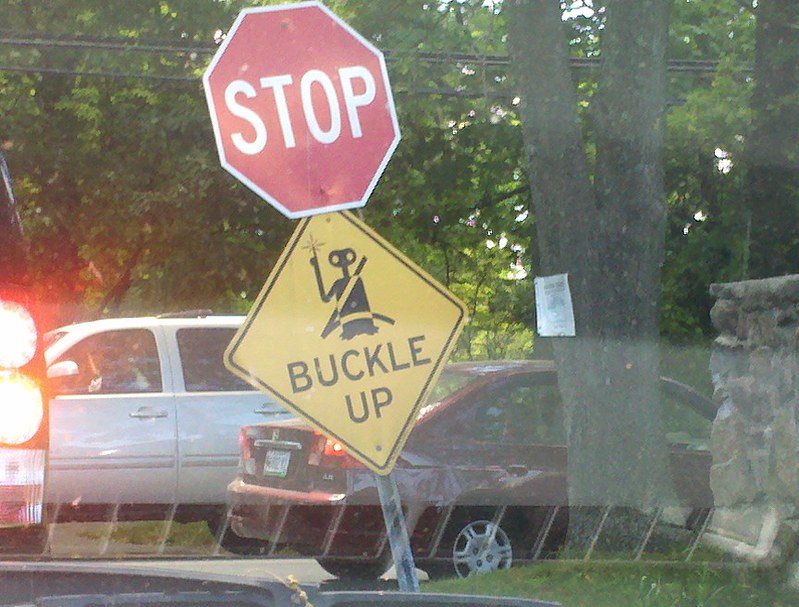This detailed photograph captures an outdoor traffic scene, likely taken from inside a vehicle approaching a T intersection. Dominating the image is a standard red octagonal stop sign displaying the word STOP in white, uppercase letters. Beneath it, a quirky diamond-shaped yellow sign features a black silhouette of E.T., the extraterrestrial. E.T. is depicted with a seatbelt strapped across his body, holding up a glowing finger in his iconic pose, accompanied by the words "Buckle Up" in black text below.

In the foreground, the viewer's vehicle is braking, as indicated by the car in front of them on the left. To the right, a large tree marked with what appears to be a lost dog poster stands near a masonry stone wall which either ends or turns the corner. The background reveals additional traffic, including a burgundy car and a silver or white truck, reinforcing the bustling environment. Further details include green-leaved trees and what seems to be part of a backlight of another car, as well as a peculiar, possibly reflective object on the left side that could be mistaken for a light or emergency vehicle indicator.